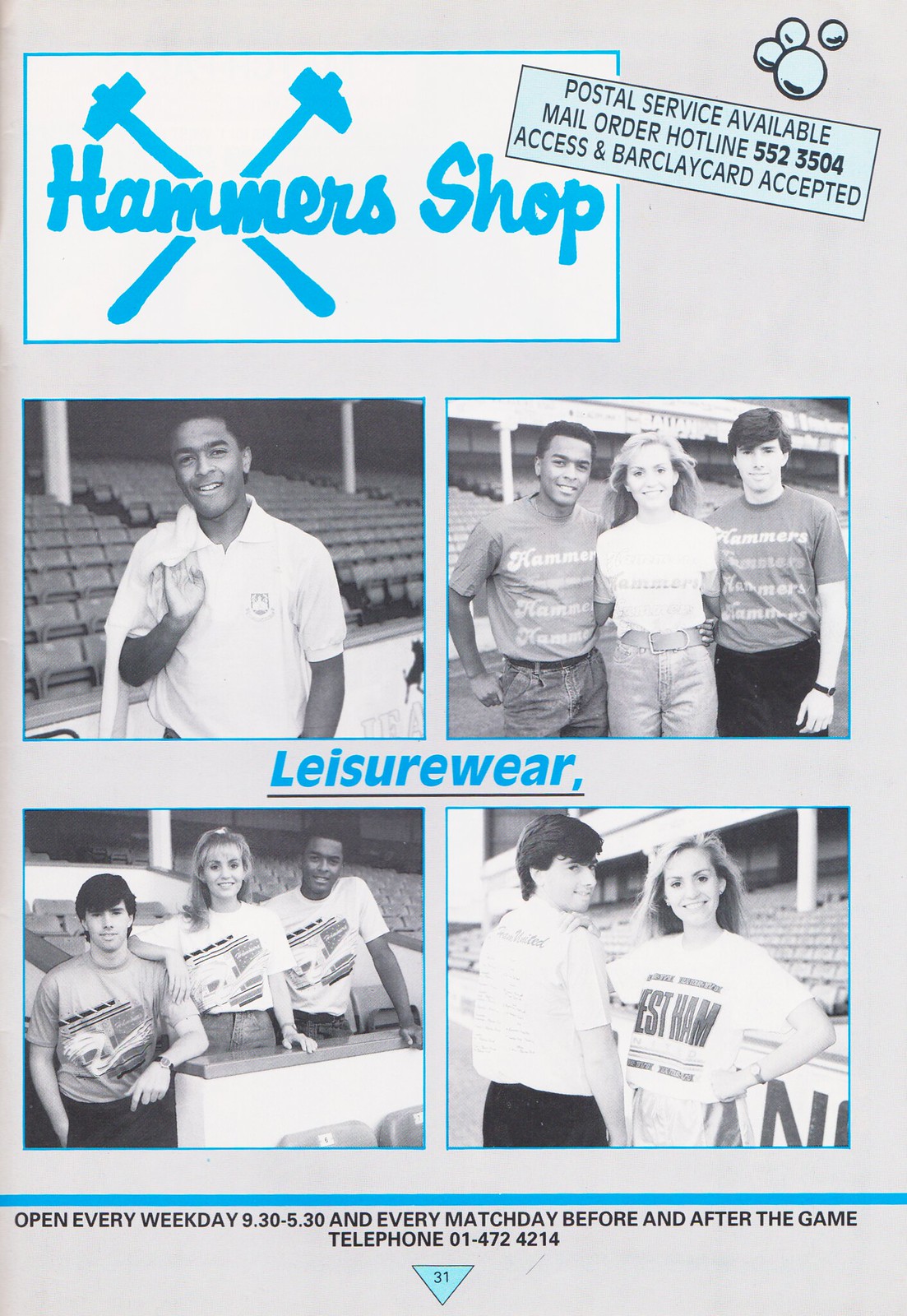This image is a black-and-white advertisement with blue accents, prominently featuring the Hammer's Shop. At the top left, inside a white rectangle with a blue border, the name "Hammer's Shop" is displayed in blue font, accompanied by a graphic of two crossed hammers. Adjacent to this, a light blue tilted rectangle announces, "Postal Service Available - Mail Order Hotline 552-3504; Access and Barclay card accepted," with stylized bubbles nearby.

The advertisement showcases four black-and-white photographs. The first two images at the top feature an African-American man in a lightly-colored shirt staring directly at the camera, and another image showing a girl flanked by two men. Below these images, the caption "leisure wear" appears in blue text.

At the bottom, two more photographs are displayed: one depicting a girl standing between two men, and another showing a man facing away from the camera but looking back, alongside a girl facing the camera. 

Additionally, the ad provides store details, stating it is open every weekday from 9:30 to 5:30 and on every match day before and after the game. The telephone number for inquiries is also listed, enhancing the advertisement's informative appeal.